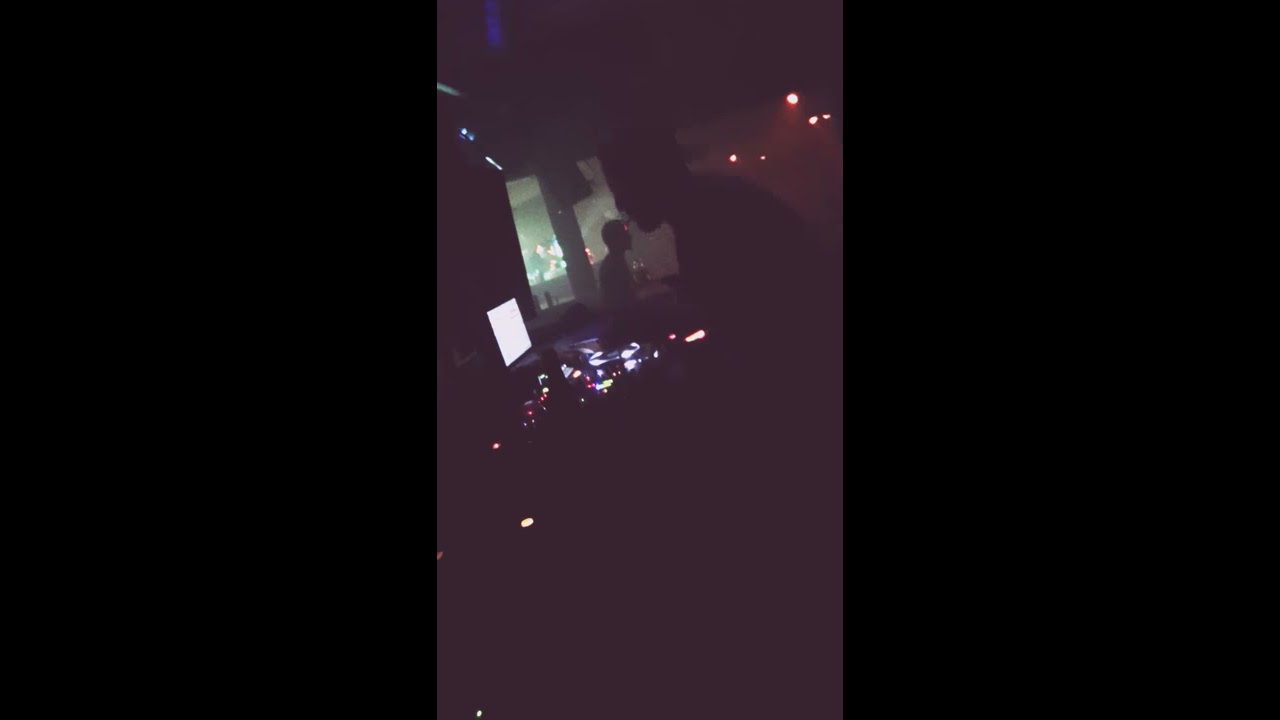The image captures a dark, nightclub scene dominated by shadows and minimal lighting. In the foreground, a man, indistinct in features but distinguishable by a backward hat, operates a DJ station with a small, white-lit monitor. Illuminated by flickering lights from the DJ equipment, he appears engrossed in his task. A lit cigarette adds a dim glow, barely highlighting his presence. Behind him, another man lingers in the shadows, further suggesting the presence of a lively, albeit unseen, crowd enveloped in the dark ambiance. Small orange and green lights from the equipment and background elements punctuate the overall obscurity, contributing to the mysterious and energetic atmosphere of the club.